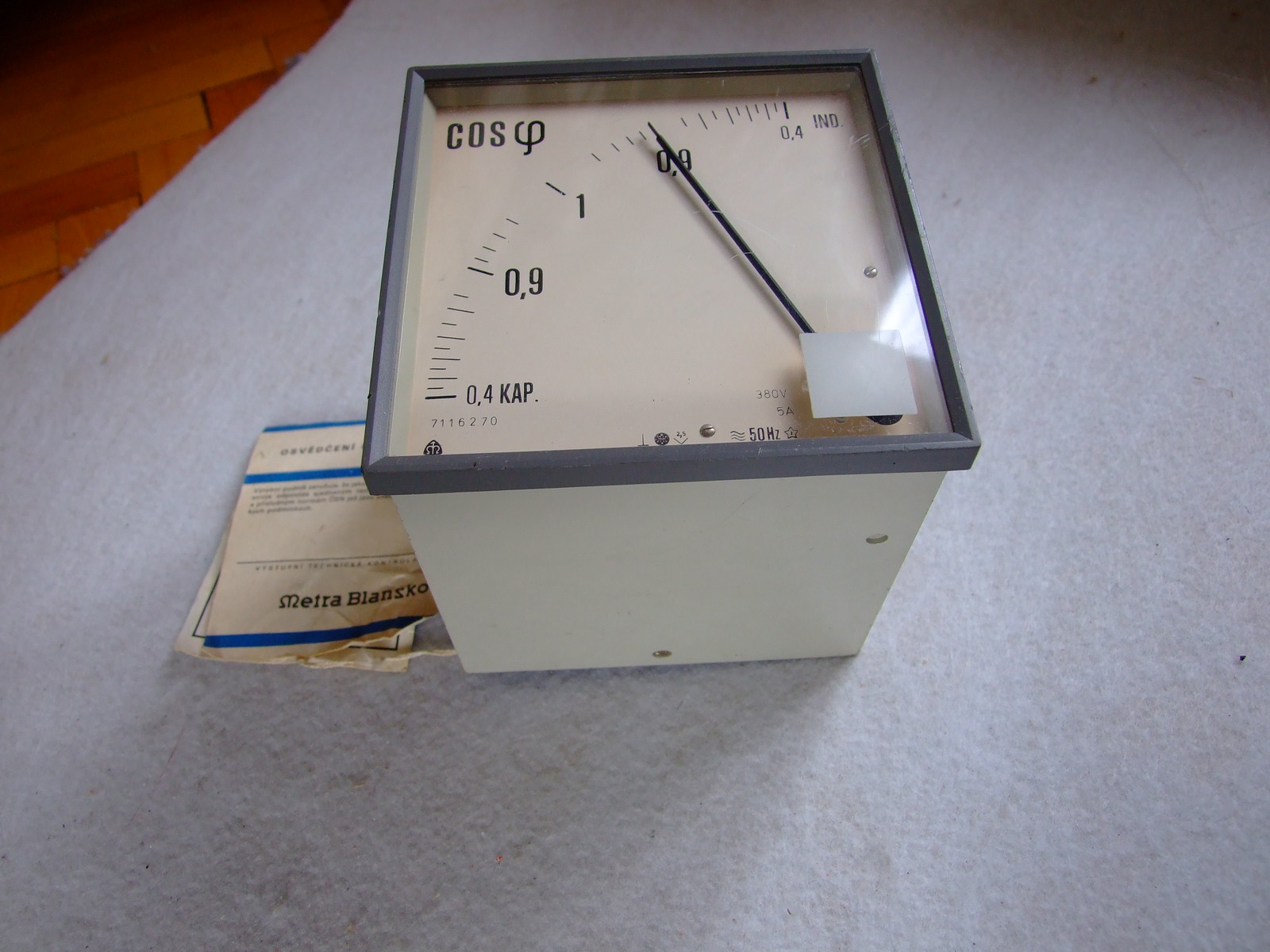The photograph showcases a square-shaped item positioned against an off-white surface. The foremost side, likely the bottom of the item, is white, while the upper section, probably the front, features a sleek gray frame enclosing a glass pane. Behind the glass, a semi-circular array of dashes, each marked with corresponding numbers, is visible. A single, long black hand is anchored in the bottom-right corner, with its tip extending towards the numbered arc, indicating a reading. In the upper-left corner of the device, the letters "COS" and a wavy line can be discerned. Adjacent to this item lie several sheets of paper. The overall ensemble rests on an elevated surface, which in the upper-right corner of the image, contrasts against a background of horizontally-laid wooden flooring.